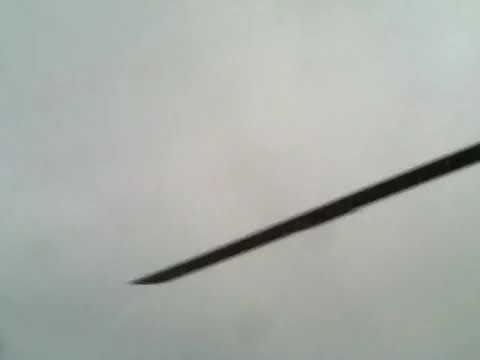The image features a close-up view of a diagonal black silhouette against a cloudy, gray background. The dark object, thin and tapering to a sharp point, originates from the upper right-hand area and extends diagonally toward the lower left. The background has a blended, cloudy-gray texture resembling an overcast sky. The contrast between the black, needle-like silhouette and the muted backdrop highlights its sharpness and angle, leaving its exact nature open to interpretation—it could be the pointed end of a needle, the edge of a blade, or even part of an aircraft wing.